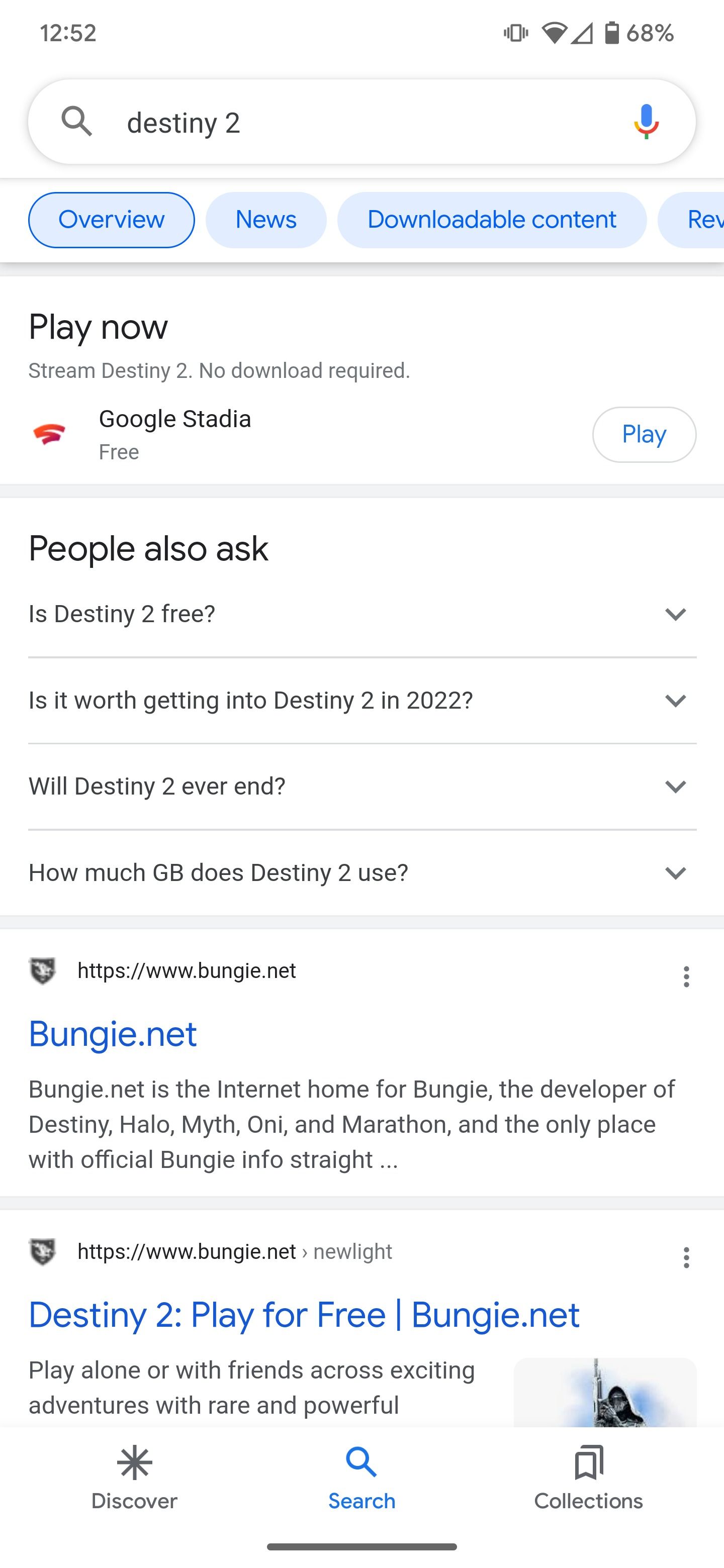A mobile screenshot from an Android smartphone displaying a Google search for "Destiny 2." The screenshot is taken at 12:52 (a.m. or p.m. not specified). In the upper right corner, there are icons indicating the phone is on vibrate, Wi-Fi is connected at about 75% strength, and mobile data connectivity is very low, around 10%. The vertical battery icon shows the battery is at 68% capacity. The interface uses a light theme. 

The search results show information about "Destiny 2," a video game. Below the search bar, tabs labeled as "Overview," "News," "Downloadable Content," and a partially cut-off option, likely "Reviews," are visible, with the "Overview" tab currently selected. The page provides a prompt to "Play now, stream Destiny 2, no download required" via Google Stadia, with a listed price of free. A "Play" button is also present beside this information.